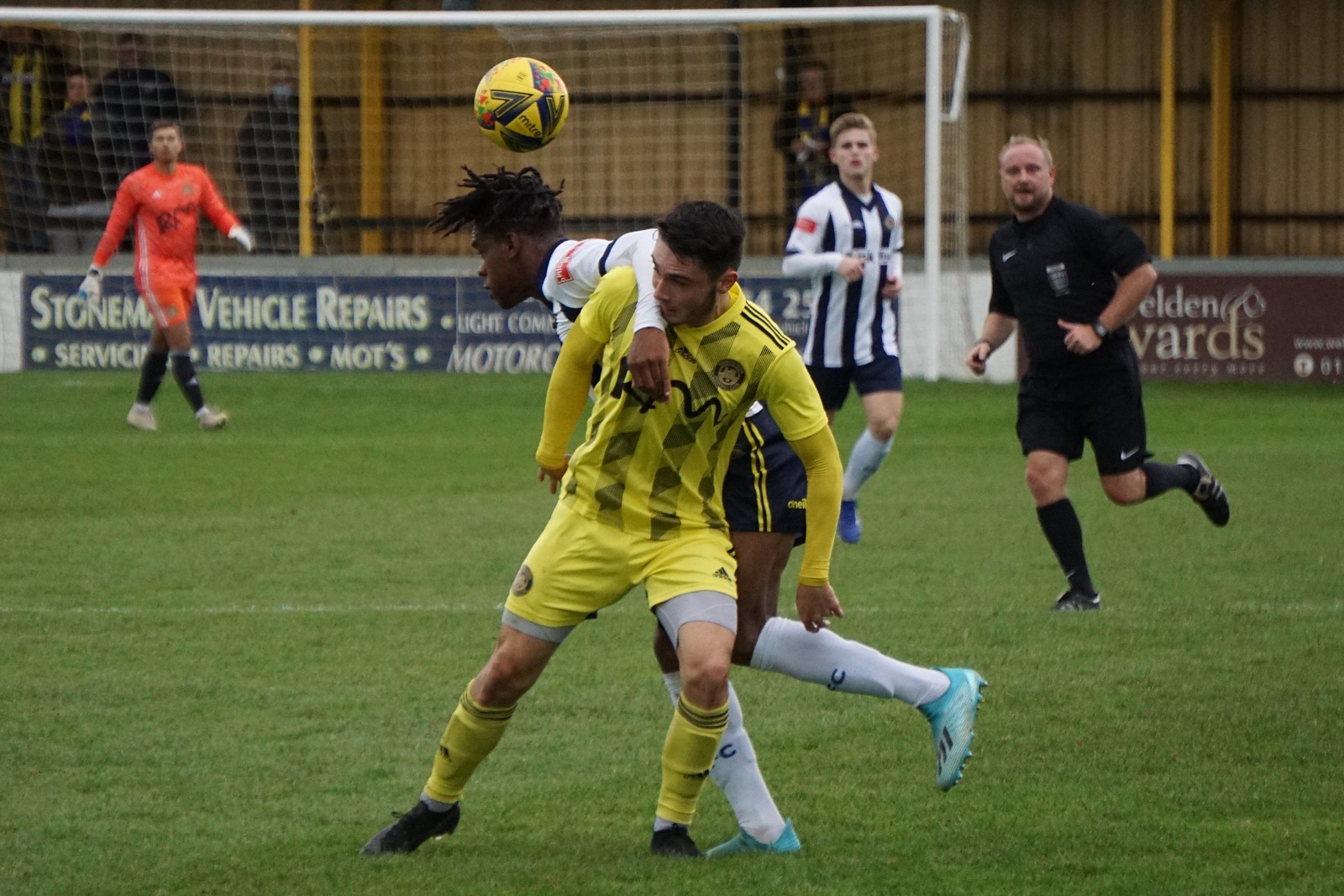In this dynamic photograph of a soccer match in progress, various players and a referee are captured in the midst of the action on a green soccer field. At the forefront of the image is a black man with dreadlocks, suspended in mid-air as he tries to head a yellow and black soccer ball. He is closely contested by a bearded player in a yellow and black uniform, who appears to be either white or Hispanic with brown hair.

To the right, a player in a black short-sleeved shirt with matching black shorts, socks, and cleats, likely the referee, is seen overseeing the game. Another player wearing a black and white striped jersey stands between the referee and the man attempting the header, possibly coordinating with the teammate on the move.

In the background, the goalie stands at attention in front of the goalposts, donned in a bright orange uniform and gloves, ready to defend. The goal posts are painted white, and beyond them, a low wall is adorned with banners advertising "Vehicle Repairs, Service Repairs, MOTs." The vivid colors of the players' uniforms and the intensity of the game create a captivating and detailed scene.